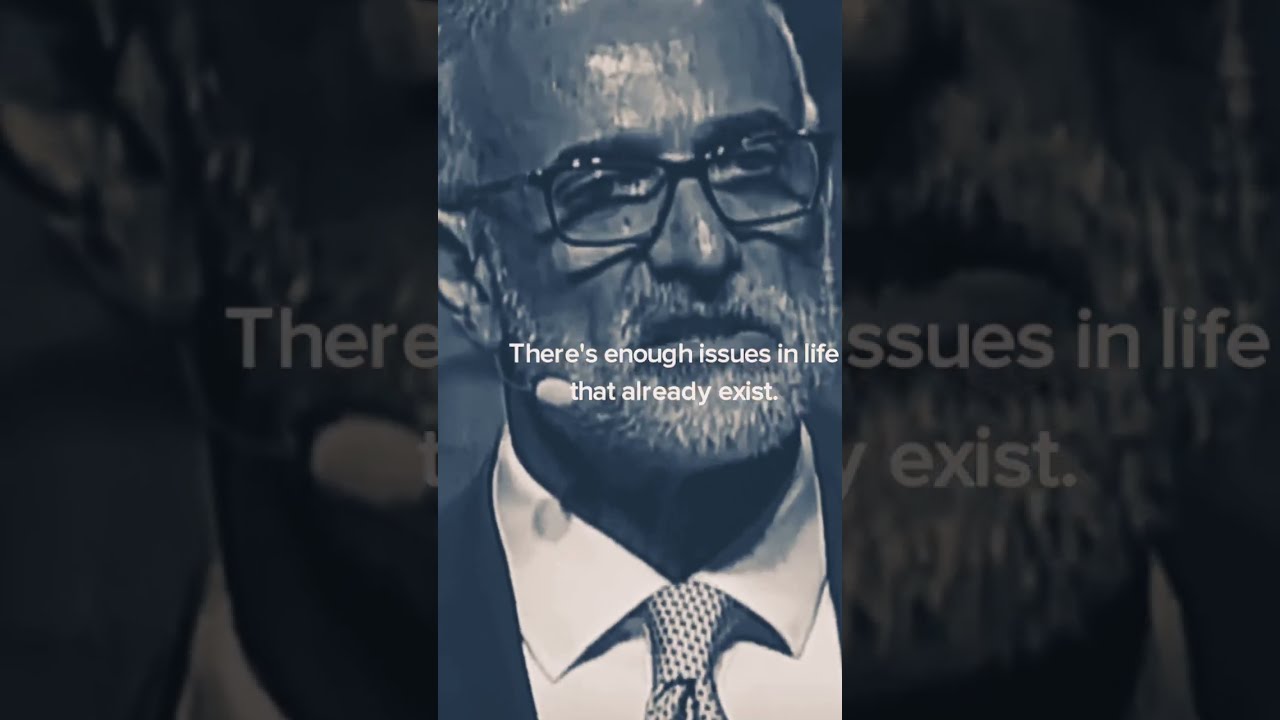The grayscale image prominently features an older, Caucasian man centered in the frame, wearing a black suit, a white collared shirt, and a dotted tie. His appearance is distinguished by a short gray beard, mustache, sideburns, and contrasting darker brown eyebrows, although the entire image is in black and white. He sports black-framed glasses and has a microphone headset with a white nib near his cheek, suggesting he is giving a presentation, similar to what one might see at a convention or keynote speech. The composition of the image is unique, with a zoomed-in version of the same photograph as its background, creating a layered effect. White text is transposed over his mouth area, reading, "there's enough issues in life that already exist." The left and right sides of the image contain fragments of the same photo, with partial text visible, reinforcing the central theme.